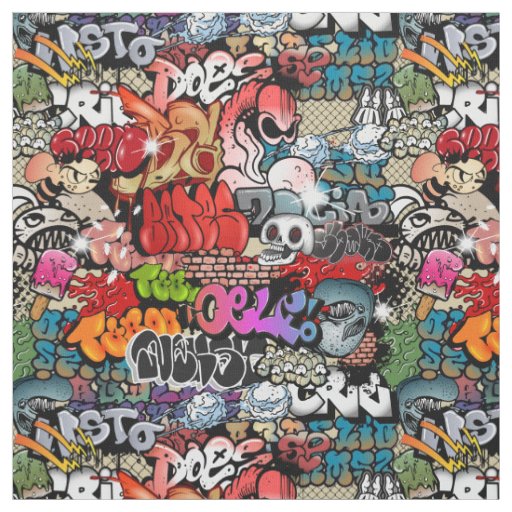The image showcases a vibrant and complex collage of graffiti, dominating the entire frame with an explosion of colors and designs. Central to the scene are chunky, colorful letters in red, purple, green, orange, black, and white, making the words difficult to decipher. Amidst the lettering, the graffiti features an array of intricate designs, including angry-looking faces of bumblebees and a prominent skeletal character with rabbit-like teeth, which appears to repeat on both the left and right sides of the artwork, creating a sense of symmetry. Noteworthy is the word "BEATS" in bold red letters positioned at the center, alongside other names such as "DOE." The dense, circular lettering style and the varied hues of red, yellow, blue, green, and black contribute to the overall chaotic yet artistic collage of urban street art.